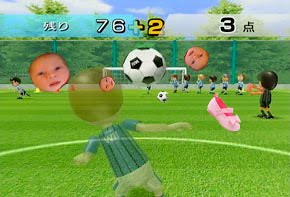The image depicts a scene from the video game Wii Sports, featuring a vibrant soccer match on a lush green field. Central to the image is a character wearing a blue and black soccer jersey with "Wii" inscribed on the back and white shorts. This character appears to be in motion, captured in a slightly translucent manner, suggesting either speed or a graphical effect. In the middle of the scene, a classic black and white soccer ball is airborne, indicating active play. In the background, additional players wearing similar jerseys and shorts can be seen, adding depth and context to the game environment. Uniquely, the image features three superimposed faces of a baby and a pair of pink ballet shoes, adding an unusual, whimsical element to the scene. At the top of the image, numerical figures "76 + 2" and "3" are visible, possibly indicating game scores or stats.